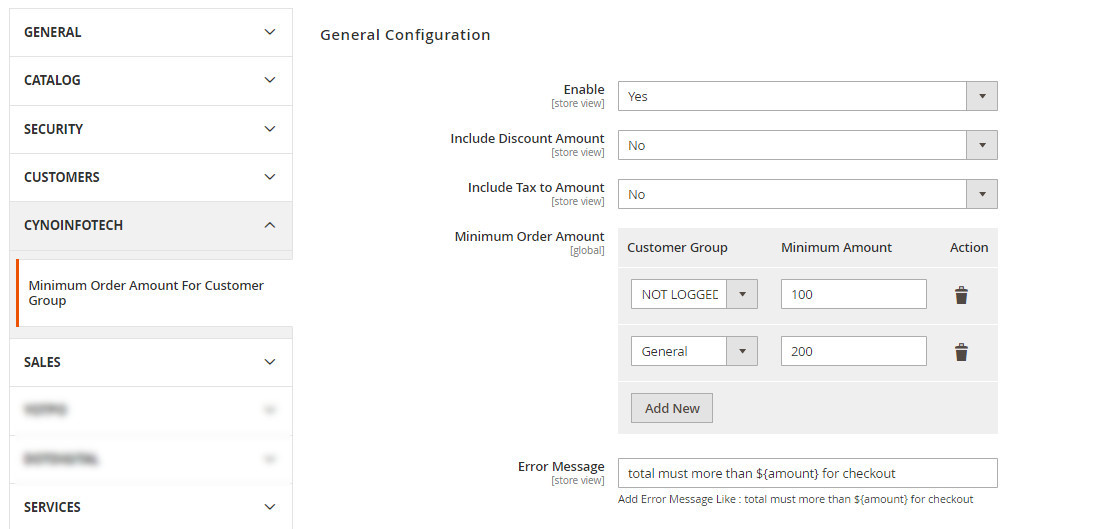This image is a screenshot of a configuration interface for an e-commerce platform, primarily focused on setting minimum order amounts for different customer groups. The layout features a vertical navigation menu on the left side with categories labeled as: "General," "Catalog," "Security," "Customers," "SinoInfoTech," "Minimum Order Amount for Customer Groups," and "Sales." 

In the central portion of the interface, under the section titled "General Configuration," various settings are detailed. These include:
- "Enable" set to "Store View, Yes."
- "Include Discount Amount" set to "Store View, No."
- "Include Tax to Amount" set to "Store View, No."
- "Minimum Order Amount" specified as "Global."
- "Customer Group" listed as "Not Logged."
- "Minimum Amount" indicated as "100."

Two lines have blurred text. Actions include a trash can icon next to "General, 200," and options to "Add New" and specify an "Error Message."

The error messages currently contain a typo, with a missing "B" between "must" and "more," both stating: "Total must more than dollar sign amount for checkout."

This screenshot is in landscape orientation and does not contain any photographic elements, people, animals, or plant life.